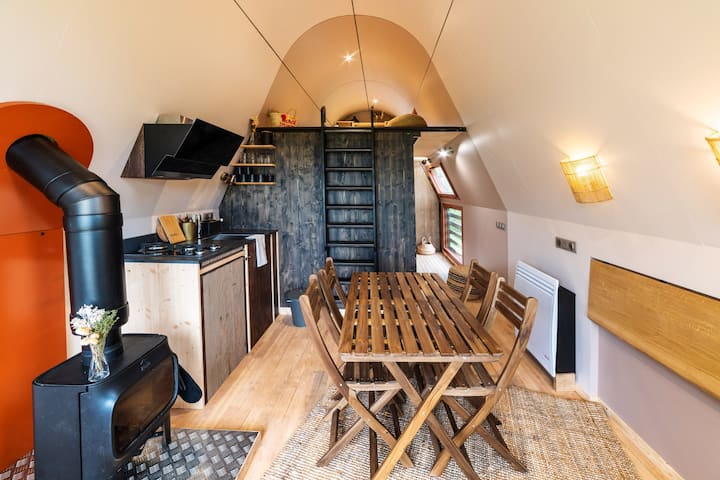The photograph captures the interior of a compact, modern micro house, characterized by its narrow space and high, domed roof which slopes inward, giving the ceiling a unique, almost gumdrop-like shape. The floor is lined with light brown wooden slats, while the walls are predominantly white with a contrasting red section behind the wood-burning stove. This black stove, positioned in the lower left corner, features a connecting pipe that leads out of the wall, and a vase with flowers rests on top of it.

Adjacent to the stove is a small kitchen area, consisting of a countertop with a two-burner stove and a sink, along with a cutting board. In the central area of the room, there is a dark-stained wooden table surrounded by four folding chairs. At the back of the room, a black wooden wall supports a ladder leading up to a loft area, which contains a bed. The right side of the wall features additional storage space constructed with wooden panels, making efficient use of the compact living area.